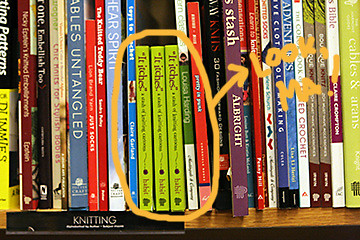The image depicts a close-up view of a bookshelf filled with various paperback books. Though many titles are out-of-focus and partly obstructed, a few legible words like "knitting patterns," "untangled," "crochet," and "spirit" suggest a collection focused on crafts. Dominating the center of the image are three shorter, lime green books titled "It Itches," aligned vertically in a neat row. An orange marker circle and arrow highlight these books with an annotation reading, "Look, Ma!" This emphasis gives a sense of admiration or excitement, possibly directed at a person named Ma. The image appears edited to draw special attention to the "It Itches" books, making them the focal point amid the surrounding, less distinct titles.